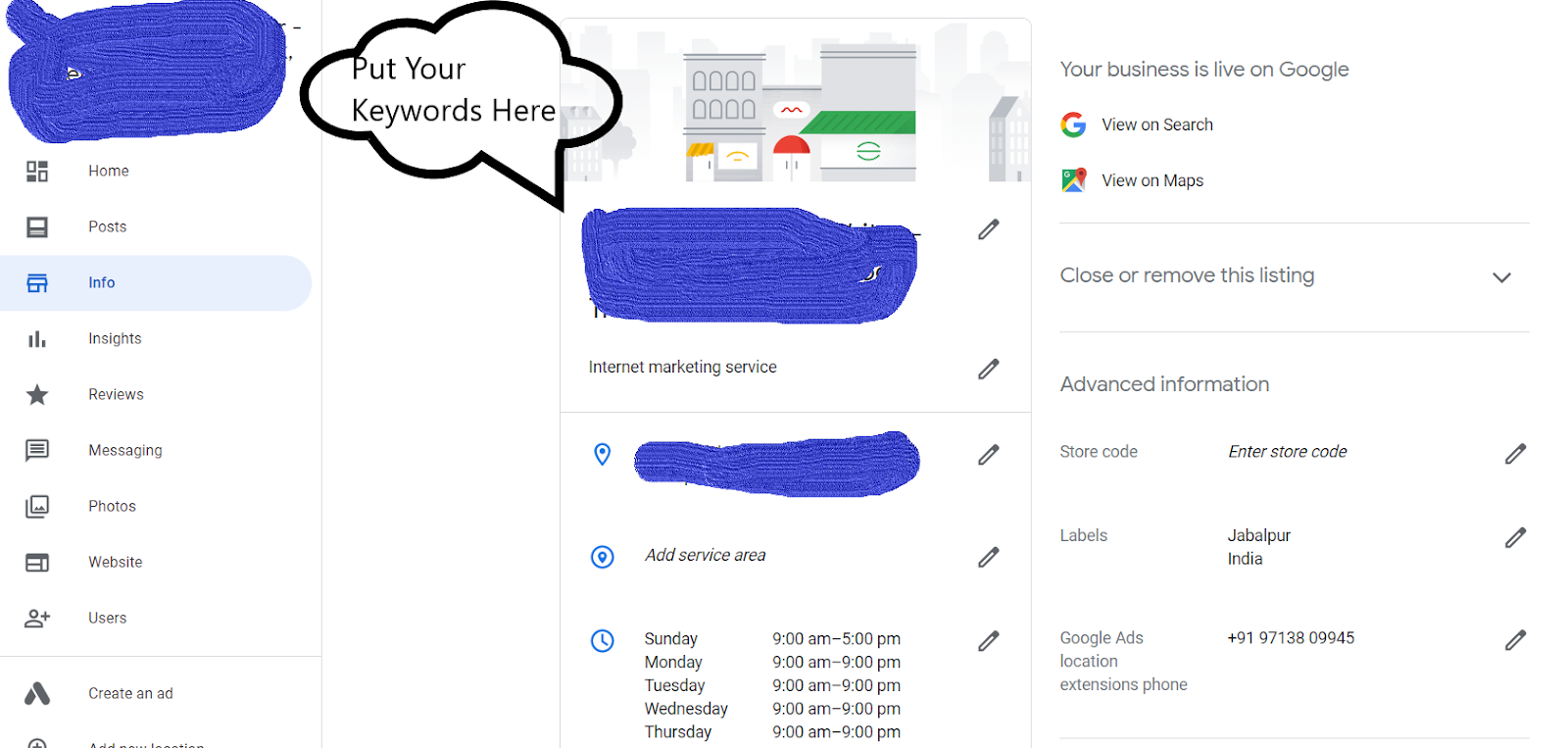The image depicts a webpage, likely a Google platform interface, although the exact nature of the site is not explicitly clear. In the upper right corner, there is a prominent notification stating "Your business is live on Google." Beneath this message are two clickable options - "View on Search" and "View on Maps." Additionally, the page features several fields that can be filled out with business-related information, each accompanied by an edit icon, suggesting that the details can be modified. A speech bubble is present, prompting users to "put your keywords here," which likely refers to SEO keywords for better visibility on search engines.

On the left side of the image, there is a vertical menu listing multiple clickable options: Home, Posts, Info, Insights, Reviews, Messaging, Photos, Website, Users, and more, indicating that users can navigate different sections to manage various aspects of their business's online presence. The central part of the page displays what appears to be an overview of business buildings or relevant visuals associated with the business. The overall design indicates an interactive dashboard aimed at helping businesses manage their Google listings efficiently.